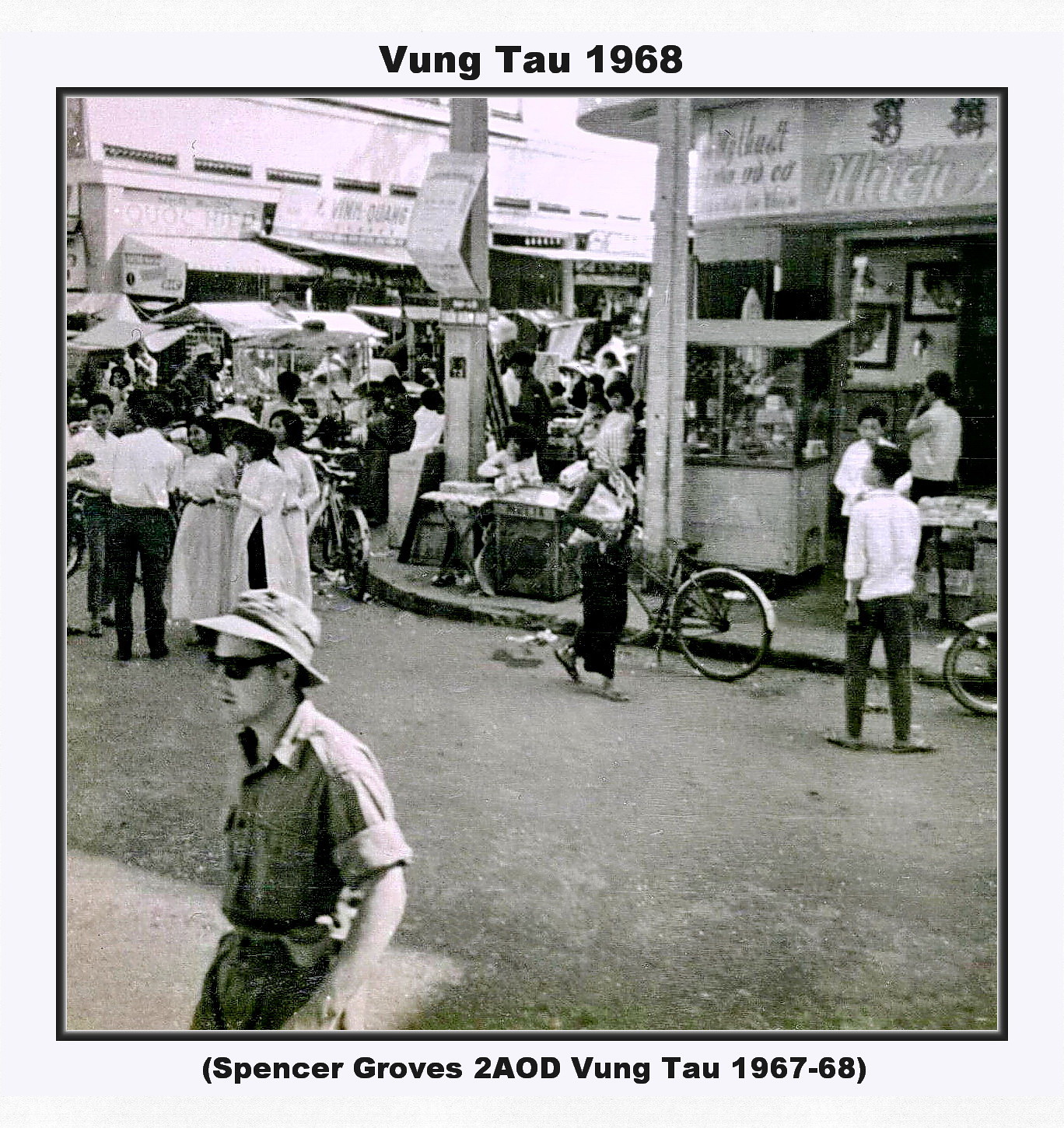This black-and-white photograph captures a bustling marketplace scene in Vung Tau, Vietnam, from 1968. The image, bordered in white with a thin inner black border, features hand-lettered captions: "Vung Tau, 1968" at the top and "Spencer Groves, 2AOD, Vung Tau, 1967-68" at the bottom. The street is lined with various buildings and sidewalk vendors, hinting at a vibrant local commerce. The unfinished roadway is devoid of markings, and numerous people, mainly appearing to be local Vietnamese in traditional attire such as long skirts and belts, populate the scene. Bicycles are prominently scattered throughout the area, emphasizing the era's mode of transportation. In the foreground, a Caucasian gentleman, distinguishable by his rolled-up sleeves, safari-style hat, and black sunglasses, contrasts with the predominantly local populace. The photograph effectively portrays the daily life and cultural crossroads of Vung Tau during the late 1960s.